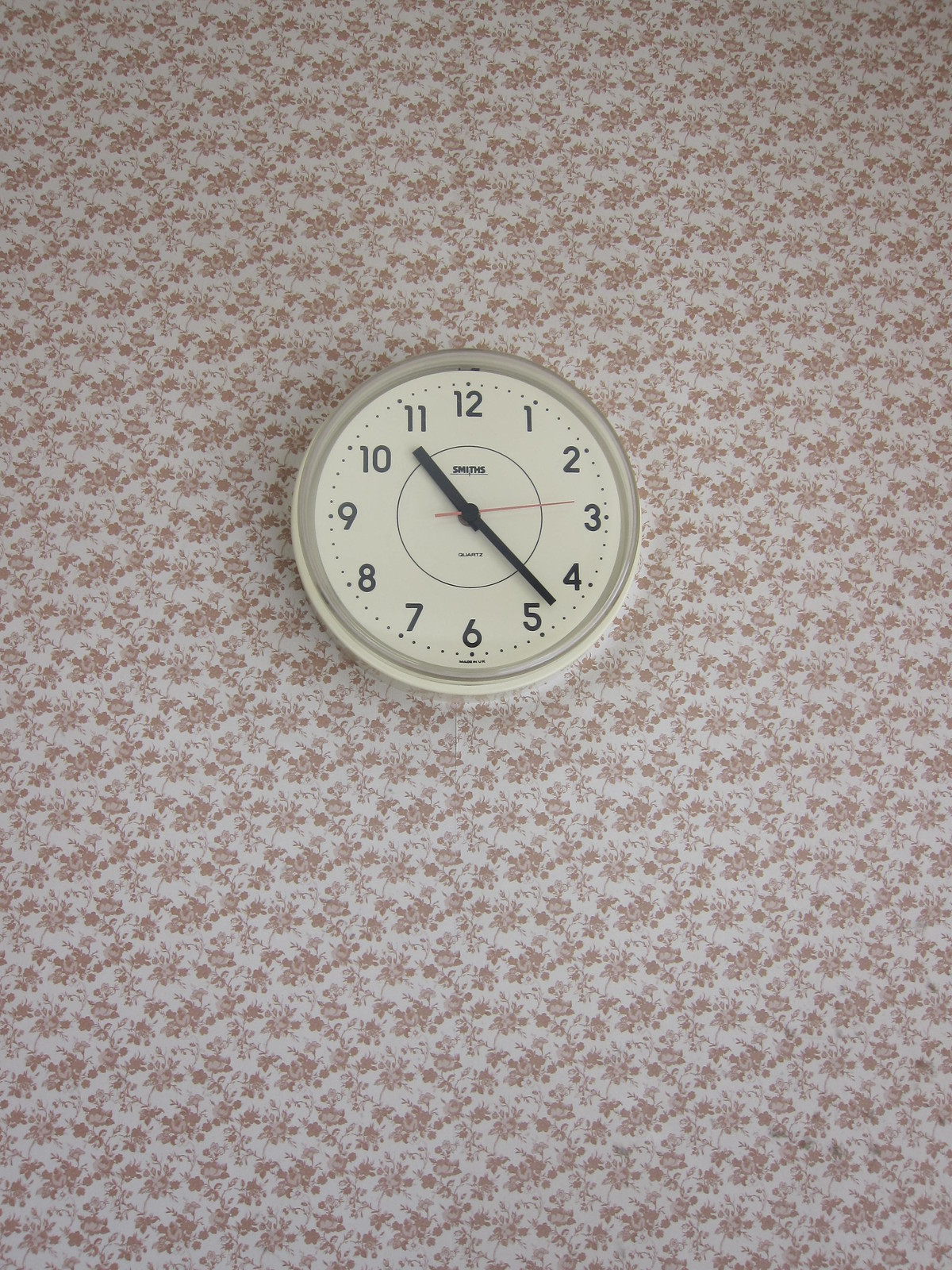This photograph captures a wall-mounted clock set against a vibrant backdrop. The wall is adorned with a red floral patterned wallpaper on a pristine white background, which provides a striking contrast to the clock itself. The clock features a predominantly white face, rimmed with a sleek silver or gray border. Bold, black standard numerals mark the hours, clearly visible against the white clock face. At the time the photograph was taken, the clock reads 10:23. Adding a subtle pop of color, the red seconds hand is positioned just above the three on the clock face, ticking away with precision.